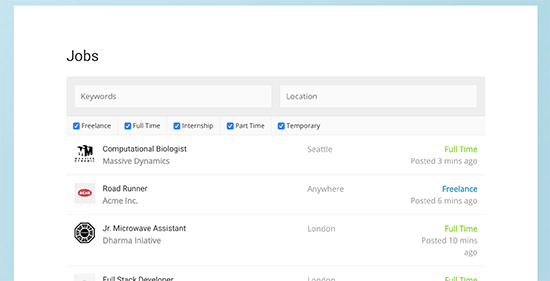The image depicts a cropped webpage with the title "Jobs" prominently displayed in the upper left-hand corner in black font. The webpage features a clean white background with a light blue border; the border is noticeably thicker on the left and right sides, and thinner at the top. The bottom part of the page appears to be cropped, as indicated by the cut-off text and absence of the blue border there. 

Below the "Jobs" title, there's a search section consisting of two input fields where users can type in keywords and locations. The input fields are set against a lighter gray background. Underneath the search fields, there are options for job types, allowing users to filter by freelance, full-time, internship, part-time, or temporary positions.

Three job listings are displayed that match the provided search criteria:
1. Computational Biologist at Massive Dynamics
2. Roadrunner at Acme Incorporated
3. Junior Microwave Assistant at Dharma Initiative